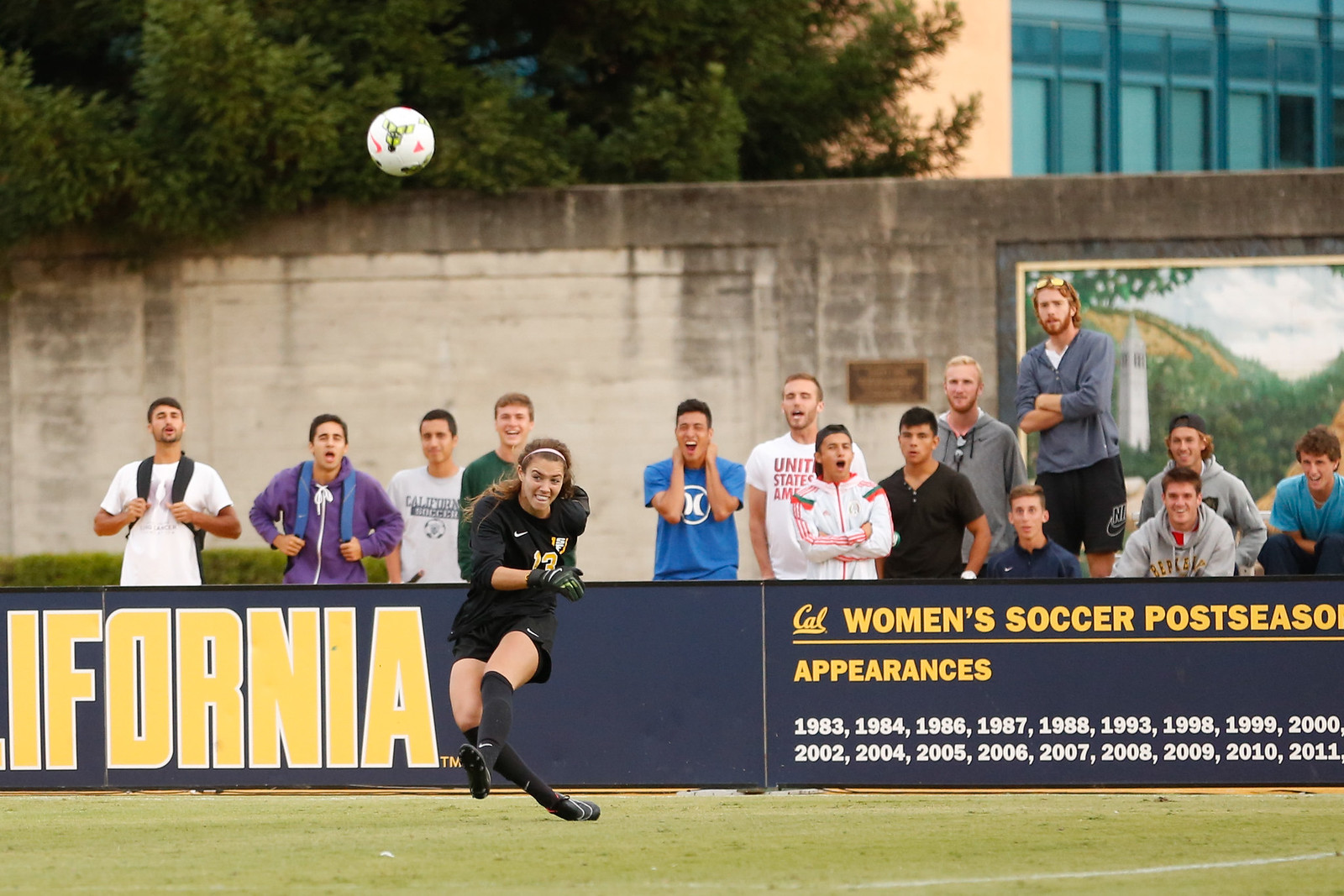In this vibrant outdoor scene, the image captures a grassy soccer field under the midday sun. Central to the composition is a woman energetically chasing a soccer ball, illustrating dynamic motion. Behind her, a wall adorned with the text "California Women's Soccer Postseason Appearances," lists various dates, serving as a testament to the team's achievements. Beyond the wall, a crowd of spectators is assembled, their figures a mixture of colors, including dark blue, light blue, purple, pink, and orange. Additionally, an artistic piece, possibly a mural, and a building are visible in the upper right corner, adding depth to the background. The overall ambiance exudes a lively outdoor sporting event, marked by the presence of enthusiastic spectators and the dedicated athlete at the image's focal point.